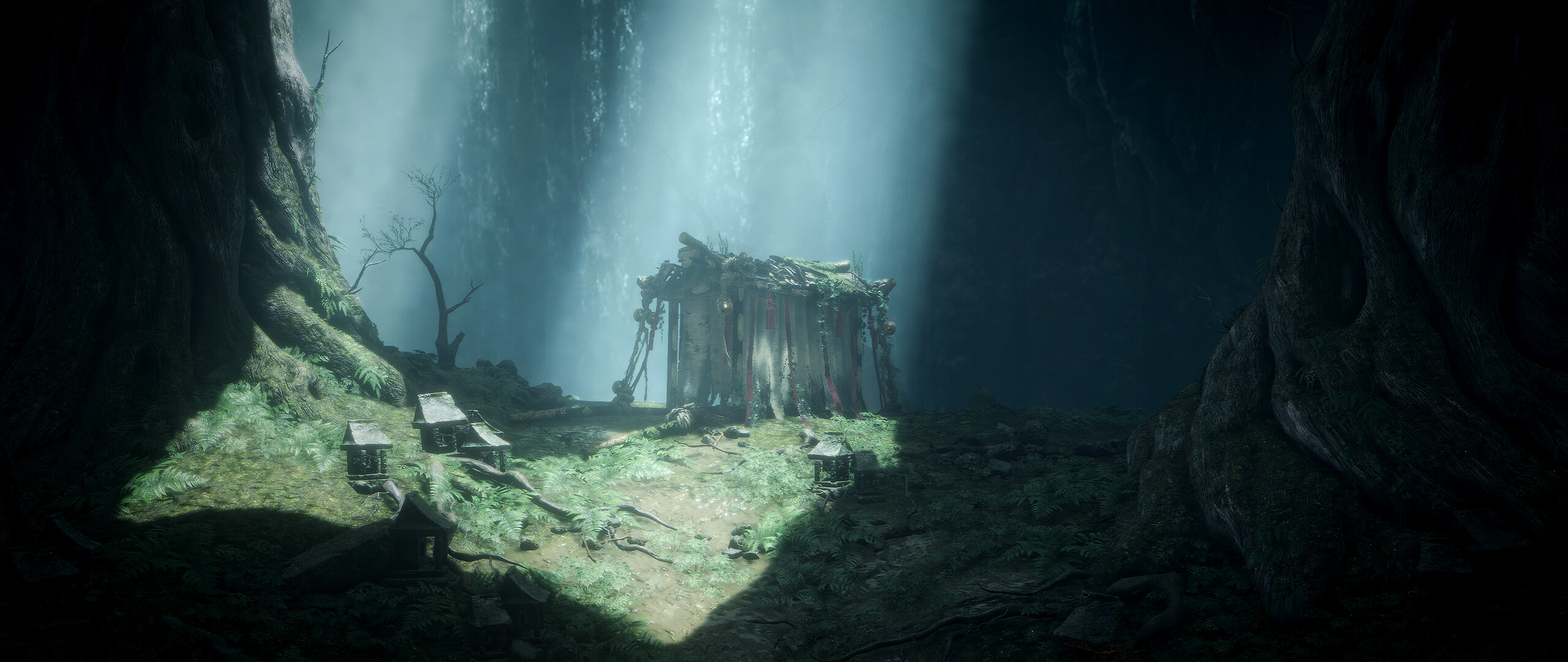The image, which appears to be computer-generated or a painting, showcases a rugged little shack as its central focal point. This main structure, seemingly built from forest resources, stands illuminated by a beam of sunlight piercing through the dense canopy of a deep forest. The surrounding scene exudes an eerie, whimsical feel due to the contrasting play of light and dark. The right third of the image, and the left edges, are enveloped in darkness, further enhancing the mystical atmosphere. The foreground features patchy grass and an assortment of smaller bungalow-style shacks and fairy houses, some adorned with pink or purple flags and intertwined with vines. Large trees tower in the background, partially shrouded in the shadows. In addition, a tree trunk with branches and a series of small birdhouses are highlighted. The right side also hints at the presence of waterfalls and a mountain edge, adding depth and enchantment to the seemingly magical forest setting.